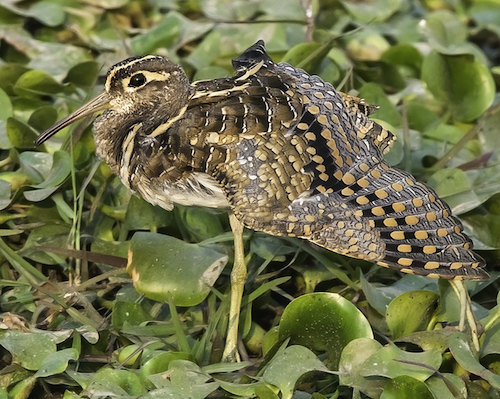The image captures a small, intricately patterned shore bird standing gracefully on one leg amidst lush greenery and water plants. The bird's plumage is a rich tapestry of colors and patterns: its overall feathers are light brown with darker brown and black accents, and its wings display a striking mix of yellow circles and black stripes reminiscent of butterfly wings. A vivid yellow stripe runs from the top of its brown head down its neck, complementing the yellow oval around its black eye. This bird also features white chest feathers and a distinctive long, thin beak that transitions from gray at the base to black at the tip. The bird's long, greenish-yellow legs are partially submerged in water plants, possibly hyacinths, while its right wing is slightly open, revealing the beautiful array of colors. The scene is a close-up, naturalistic setting with no visible forest or broader environment, highlighting the bird's detailed and vibrant plumage against a backdrop of varied green leaves and stems.